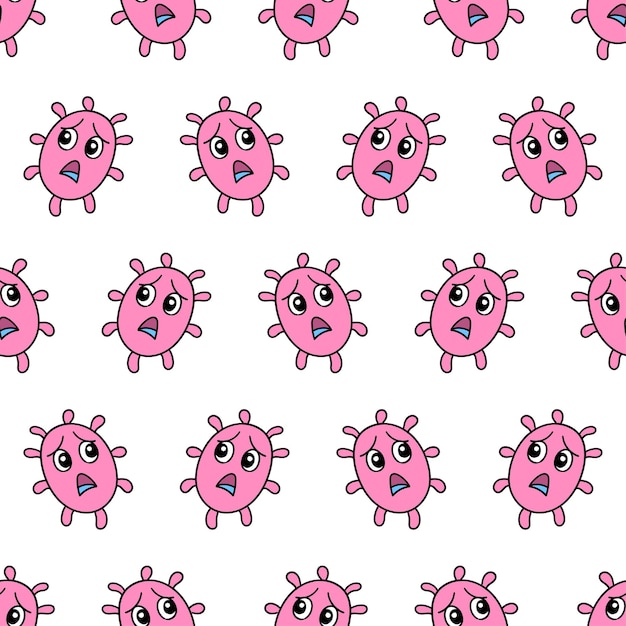The image displays a repeating pattern of pink cartoon microorganisms on a white background. Each microorganism is a pink oval shape with nine stubby tentacles protruding from all around its body, resembling an amoeba form. They have black eyes, furrowed eyebrows, and open mouths with blue-colored tongues, giving them a nervous and upset expression. The pattern alternates the direction in which the microorganisms face, creating a mirror image effect. This layout forms five rows, where each row contains four to five of these pink beings, intensifying the sense of an unsettling yet whimsical repetition.